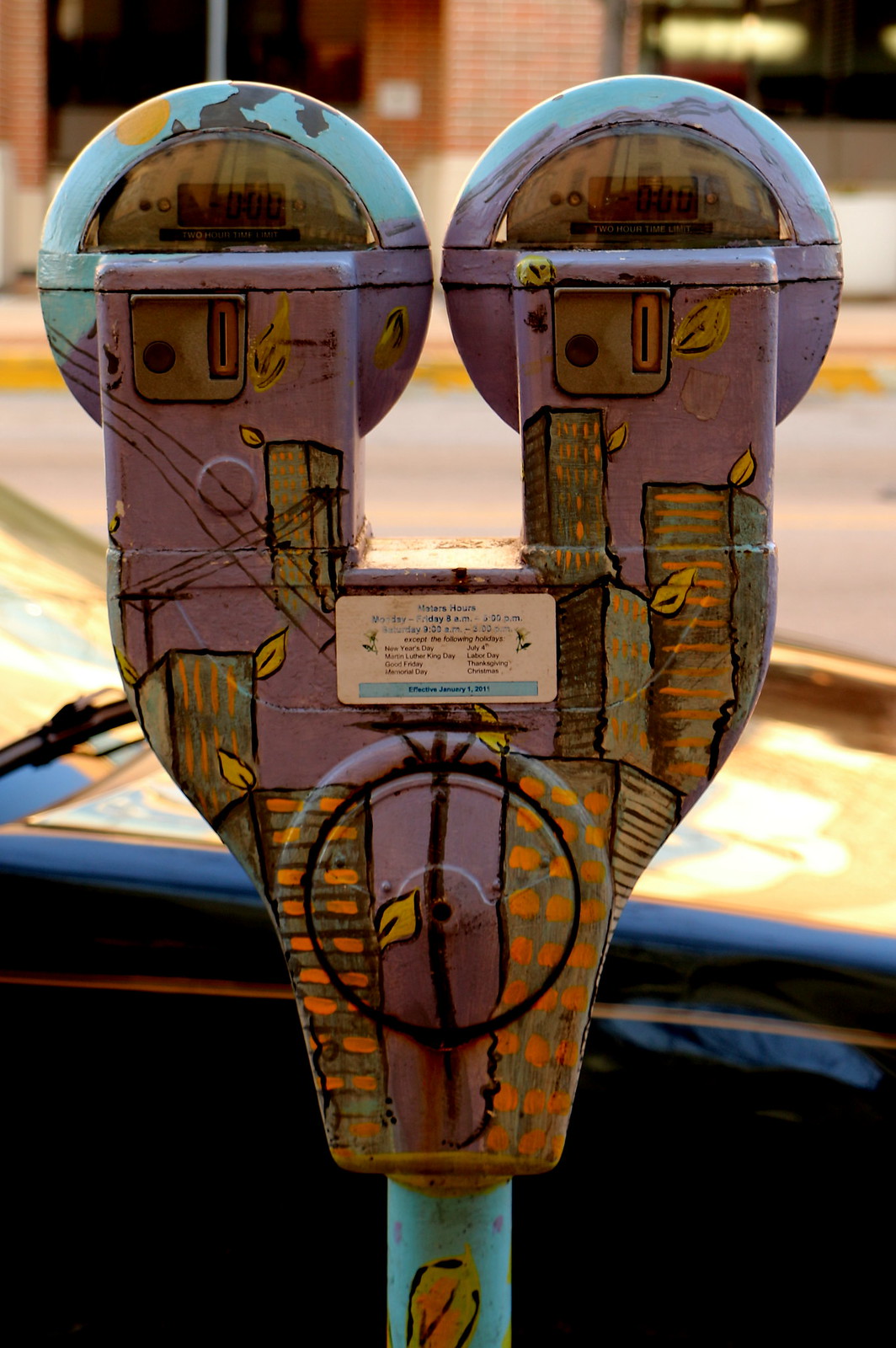This photograph showcases a vibrantly painted double parking meter set against an urban backdrop. The parking meter, designed for two parking spots, features a meticulously hand-painted design. The tops of the meters are a vivid blue, adorned with images of clouds, mountains, and the sun. Moving down, the meter displays are visible with zero time remaining. The upper portion of the meter transitions into a light purple, filled with a skyline of grey and orange city skyscrapers with brightly illuminated yellow windows. Scattered throughout this section are falling yellow leaves, with one descending all the way to the light blue pole that supports the meter.

The background reveals a typical city street with visible brick buildings and a sidewalk. A dark blue or black car with a hood that hints at a yellow tint rests beside the meter, showcasing details like an orange strip and wipers on the windshield. Further elements include electricity towers and wires painting an intricate cityscape. The scene is rich with artistic flair, blending urban functionality with creative aesthetics.